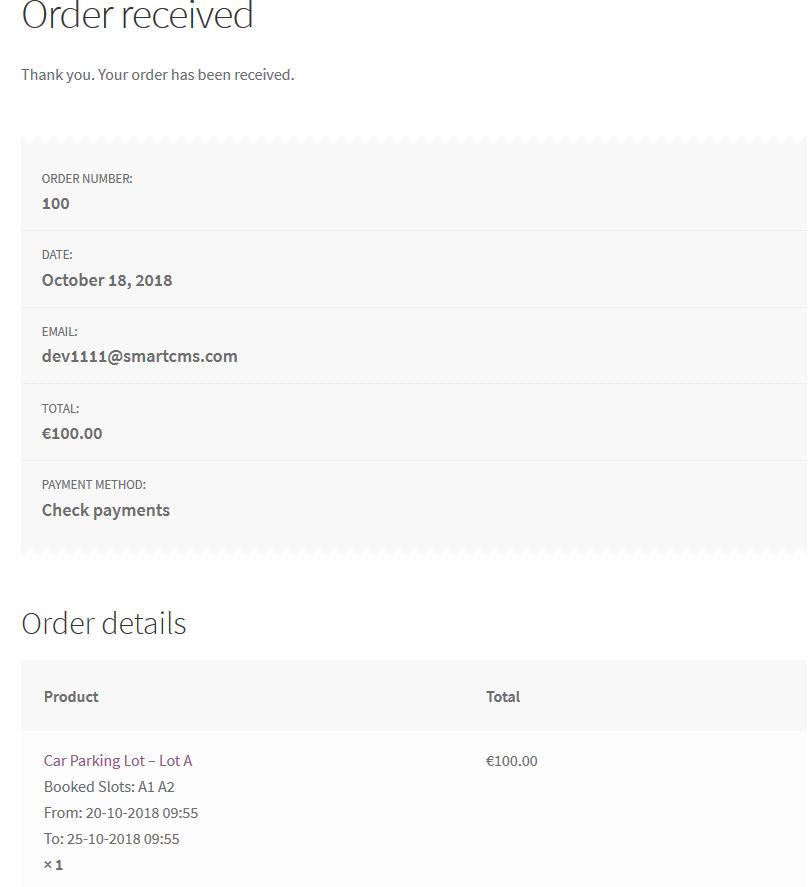This image depicts a receipt for an online order, marked by a heading that reads "Order Received." Beneath this heading, a confirmation message says, "Thank you, your order has been received." 

In a gray box, the receipt details essential order information, including the order number, date, customer email address, total amount, and payment method, which is specified as check payments.

Below this information, a white section introduces a new heading in gray, "Order Details," followed by a darker gray section outlining specifics. It lists "Product" and "Total" in bold. The product is identified as "Car Parking Lot A" in purple text, with slot bookings at A1 and A2. The dates of use are also provided but are not specified here.

The receipt further notes a total amount of 100.00, displayed with a European currency symbol instead of a dollar sign, indicating the cost of the parking slots. Beyond the specifics of parking in slots A1 and A2, no additional details are provided.